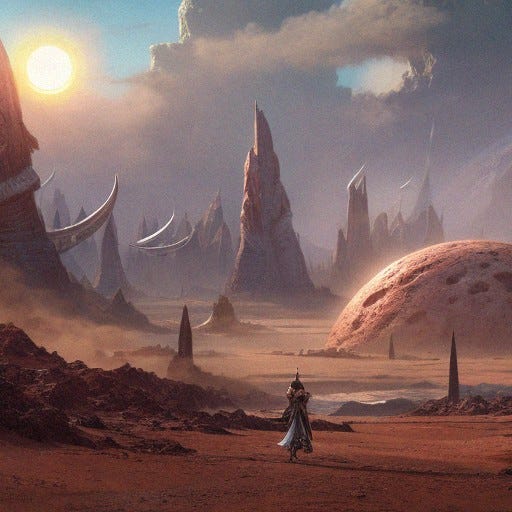This square digital illustration depicts a fantastical, science-fiction landscape on an alien planet. Dominating the foreground is a reddish-brown sandy terrain that covers the bottom 20-25% of the image. In the center, a solitary figure, roughly one-eighth the height of the image, walks along the sand. This figure, likely a woman, wears an elaborate blue dress with a thick collar; the dress flares at the bottom, obscuring her feet, and she appears to be wearing a distinctive, pointy hat. Her shadow stretches off to the right.

On the left side of the image, there's a rocky hill-like area, while the right features a partially-visible, mushroom-shaped tree with a dark pink dome and a trunk. In the background, towering stalagmites—four to five times the height of the figure—dot the landscape, some adorned with metallic, horn-like structures.

The sky is divided dramatically: the upper left corner reveals a bright yellow sun against a light blue sky, casting a glowing aura, while the rest of the sky shifts to dark gray with heavy clouds. This otherworldly setting, complemented by small patches of exposed blue sky, gives the impression of a planet far removed from Earth.